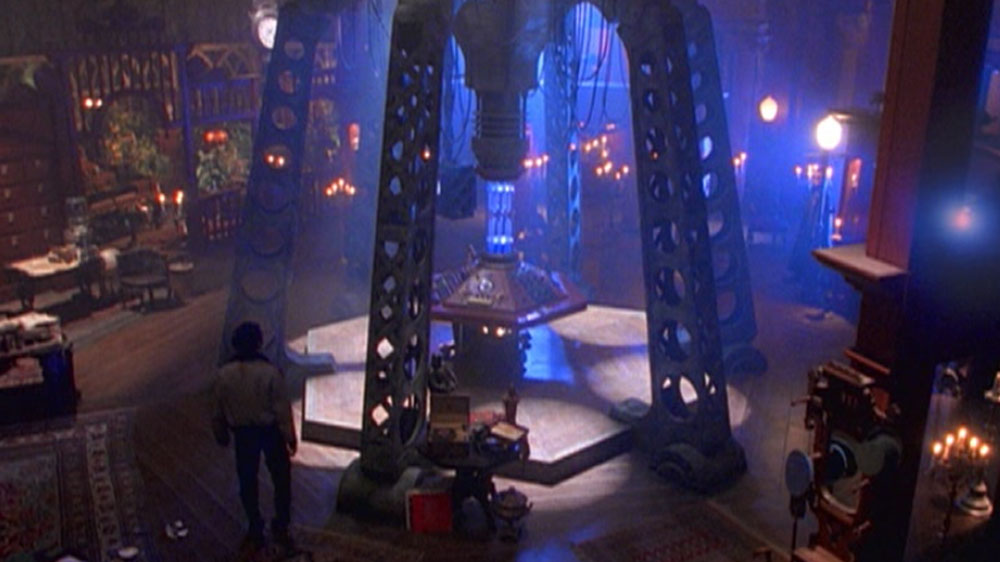In this somewhat blurry screen capture, possibly from an episode of "Doctor Who," we see a visually intricate scene set in an eclectic mix of a science laboratory, library, and dining room. The focal point of the room is a sophisticated central console, laden with advanced technological features including numerous cables and structural supports. This console is elevated on a raised platform that dominates the center of the space, exuding a sense of importance.

Surrounding this high-tech nucleus, the room is filled with a diverse array of elements: dining tables, chairs, candelabras, and a plethora of books, creating an ambiance that bridges the traditional and the futuristic. The lighting is particularly striking, with a strong, hazy blue light emanating from the central console, casting an ethereal glow that contrasts with the otherwise warm, golden wood tones and natural textures of the room's decor. 

In the background, a figure is seen entering the room. While the image's quality makes it hard to determine specifics, the individual's proportions suggest a masculine presence. They appear to be dressed in a light-colored shirt paired with darker pants. Overall, this space is a fascinating blend of technology and traditional aesthetics, visually anchored by the dynamic interplay of cool blue illumination and warm, earthy hues.